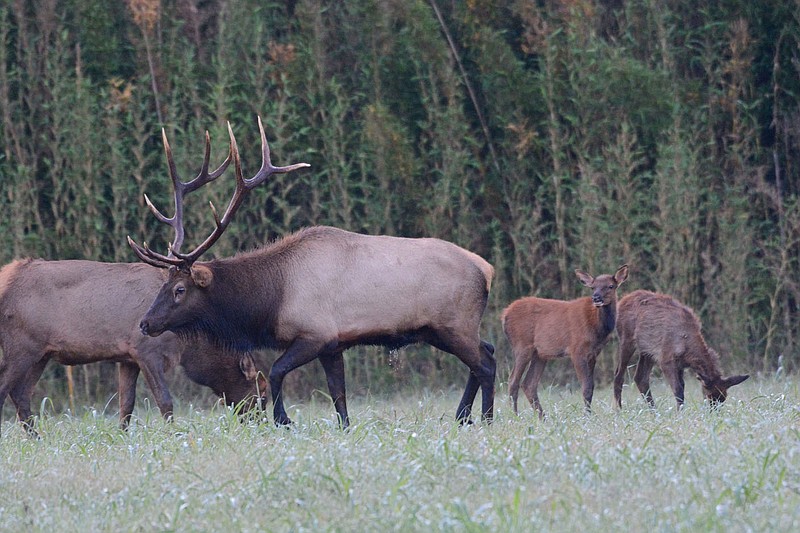This captivating photograph features a family of four deer in a lush, green meadow. The setting is serene and tranquil, with thick, wispy grass that reaches up to the deer’s legs. In the foreground, a magnificent male stag stands out with his impressive, branched antlers, dark-colored head, and contrasting grey body and black legs. To his left, another adult deer grazes peacefully, its head lowered into the verdant grass. On the right side of the image, two younger deer, possibly the offspring, are also seen, with one of them nibbling on the grass. The backdrop is a dense woodland with tall, green trees, adding depth and a sense of natural harmony to the scene. The deers appear calm and relaxed in their idyllic environment, indicating a close-knit family group.